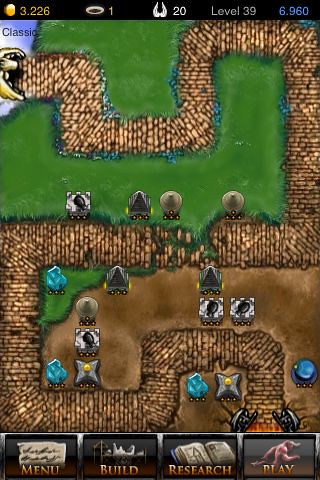This image appears to be a screenshot captured from an early era iPhone tower defense game, showcasing the distinctive portrait mode typical of that time. The game interface presents a complex, winding path made of brown bricks, resembling a labyrinth stretching from the top left to the bottom right of the screen, cutting through a landscape that transitions from grass on the top half to dirt at the bottom half. Scattered along this path are various structures, likely towers, with some marked by yellow dots indicating their level or functionality. The screenshot captures elements of the user interface (UI)—a black banner at the top displays a coin symbol with the amount 3226, the level number 39, and another indication of 6960 alongside the label "classic," suggesting this might be the game's classic mode. At the bottom of the screen, buttons for menu, build, research, and play are visible, indicating the player's control options. Additional visual elements include various tower defense weapons like an X-shaped structure, a crystal, and a cannon, with an estimated total of around 12 such structures laid out across the winding path. These details together depict a strategic setup for defending against incoming enemies in the game.